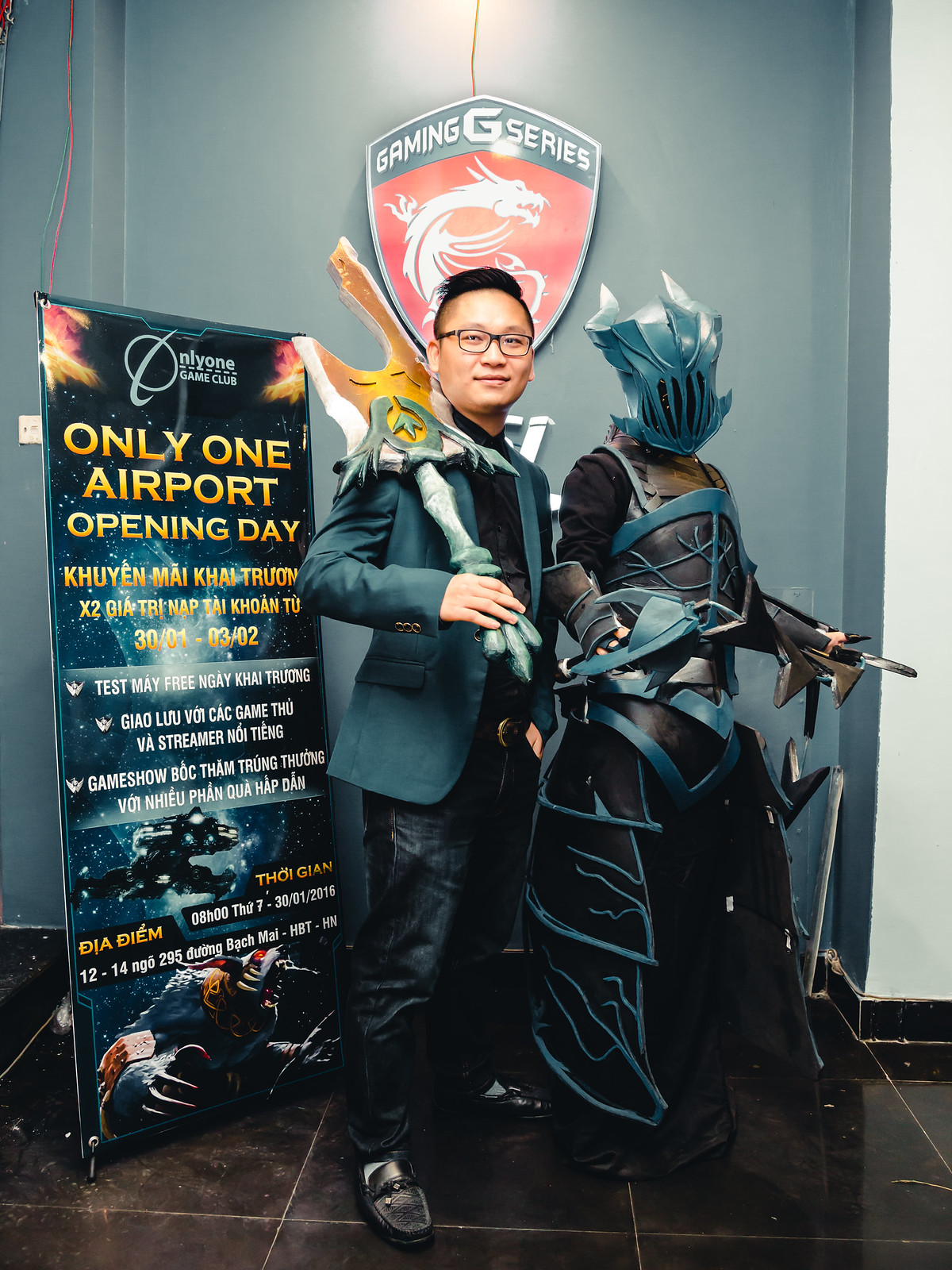A man with slicked-back black hair and black-framed glasses stands on a black tile floor against a light blue-gray wall. He is wearing a dark blue jacket, a black shirt, and dark jeans, complemented by black moccasins. The man, who appears to be Asian, is holding a play weapon resembling an axe made of a skeleton's hand. Behind him, a shield-shaped plaque with a red background and a white dragon proclaiming "Gaming G Series" hangs on the wall. To his left, a large sign reads "Nylon Game Club," and underneath it, in yellow text, it states "Only One Airport Opening Day," followed by inscriptions in another language. Posed next to the man is a figure adorned in a long robe with armor, wearing a green mask, and seemingly holding a sword, evocative of a medieval or fantastical character. The setting suggests a gaming seminar or event atmosphere.